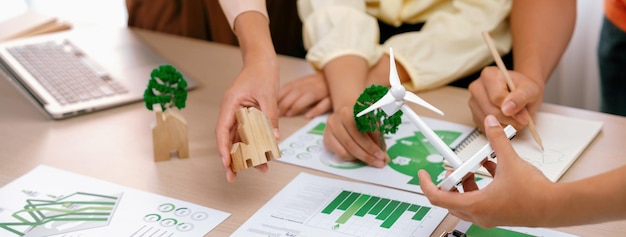A group of individuals is gathered around a wooden desk, engaged in what appears to be an architectural or environmental planning session. Various documents and diagrams are spread out on the table, all printed on white paper with green ink, including a circular pie chart, a bar graph, and other schematic drawings. The only visible parts of the people are their arms and hands, showcasing a variety of actions and items: one person on the right holds a detailed model of a wind turbine; another individual in the center holds a model of a green tree with both hands, wearing a light yellow shirt; a third person is writing notes with a brownish pencil on a spiral-bound pad; and a fourth hand is presenting a small wooden model of a building. Additionally, there is a laptop on the table, and another wooden house model is nearby, indicating a collaborative effort in planning or design.